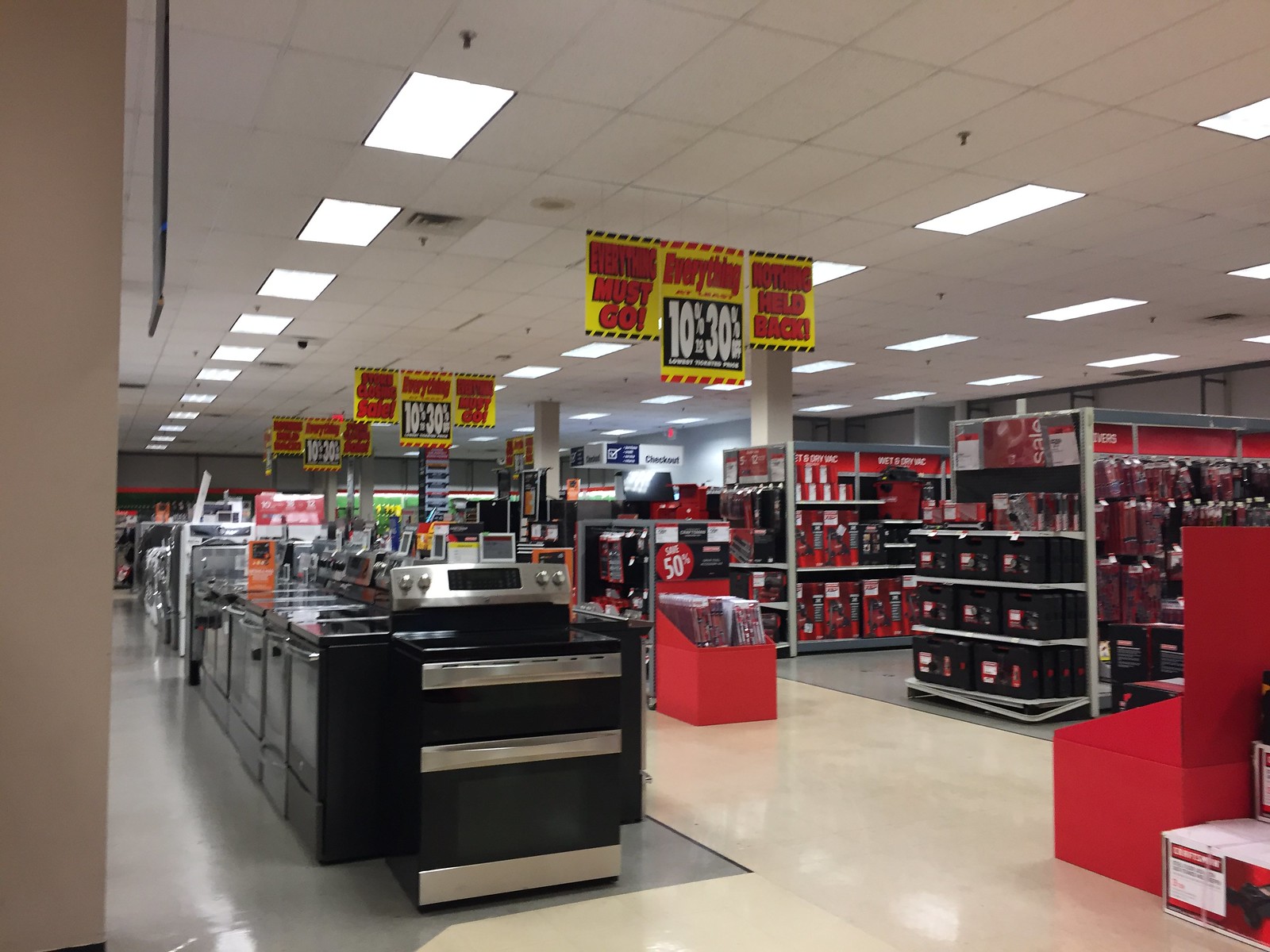The image depicts the interior of a store, possibly a hardware or appliance store, in the midst of a clearance sale. The white ceiling features rectangular designs with rows of bright rectangular lights and visible ceiling tiles and sprinkler system. Multiple yellow sale signs hanging from the ceiling, primarily on the left side, announce "Everything Must Go!" in bold red lettering with exclamation points and additional offers of 10% to 30% off. The store is organized into aisles, with a distinctive red color scheme for the aisles and displays. The store floor is a neutral white and gray, while the inventory seems to include a variety of appliances and tools. Notably, black stovetops and other appliances are visible, suggesting that the store is selling off its entire stock.